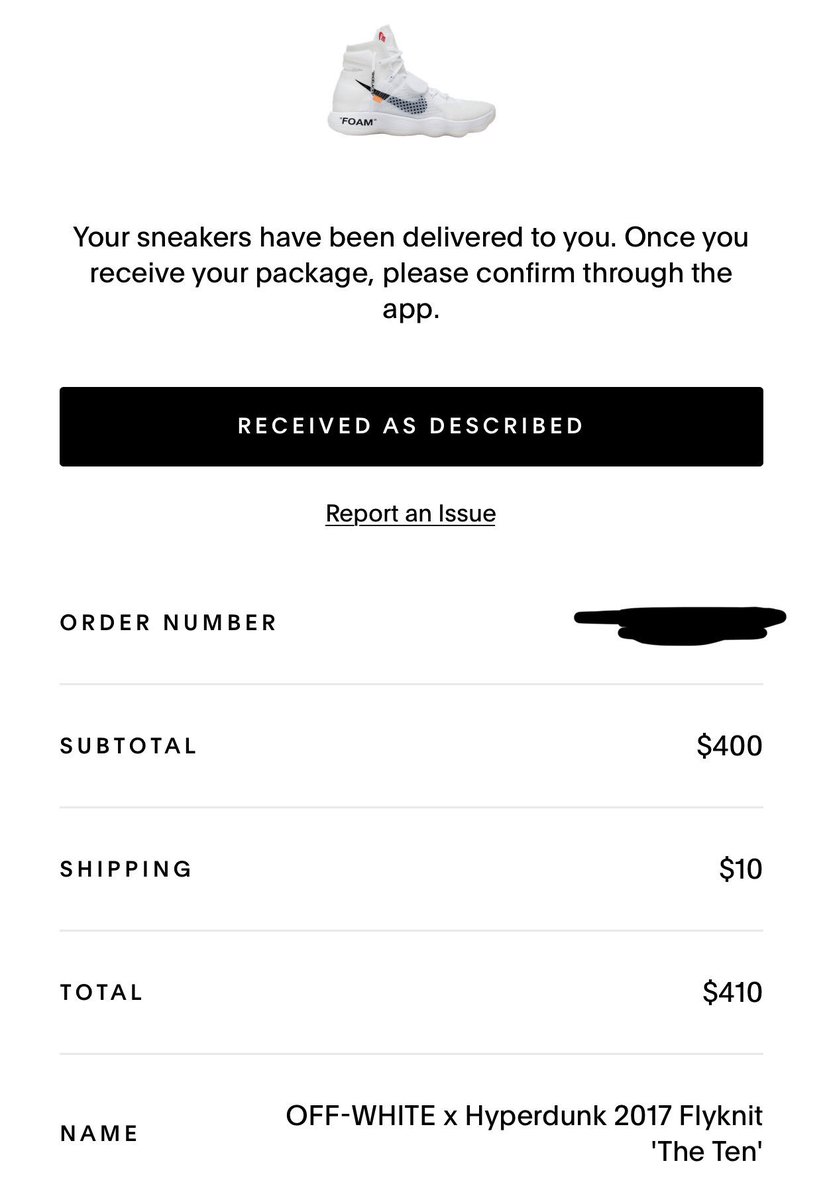On a clean, white background, the upper section features a Nike basketball shoe, positioned with its toe pointing to the right. The shoe is primarily white with a prominent black Nike swoosh on the side. Directly below the image, bold black text announces: "Your sneakers have been delivered to you. Once you receive your package, please confirm through the app."

Beneath this text is a black rectangle with two centrally-aligned options in white uppercase letters: "RECEIVE AS DESCRIBED" and, underlined, "REPORT AN ISSUE."

Following this section, bold black uppercase text stating "ORDER NUMBER" is displayed, with the actual order number obscured by a thick black line. A thin gray line separates this from the subsequent details.

The breakdown of costs is itemized as follows: 
- "SUBTOTAL: $400" in bold black uppercase letters, with a thin gray line underneath.
- "SHIPPING: $10" in bold black uppercase letters, followed by another thin gray line.
- "TOTAL: $410" in bold black uppercase letters, with yet another thin gray line below.

At the bottom, the product name is listed in bold black uppercase letters: "Off-White X Hyperdunk 2017 Flyknit 'The 10'."